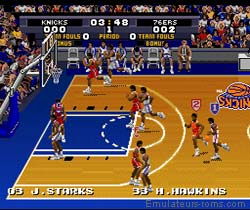Screenshot from a vintage computer basketball game showing a top-down view of the court and scoreboard. The scoreboard at the top displays "Knicks" on the left with a score of "000" and "76ers" on the right with a score of "002". The current game time, displayed in the middle, is "3:48" in the first period. Player indicators at the bottom of the screen read "03 Jay Starks" and "33 H Hawkins". At the very bottom, the website "emulators/toms.com" is visible. The court, rendered in blue and light brown, features multiple players from each team with red jerseys contrasting against white jerseys. A player with a red jersey and the number "2" is highlighted on the right, while a player in a white jersey with the number "1" is also in view.